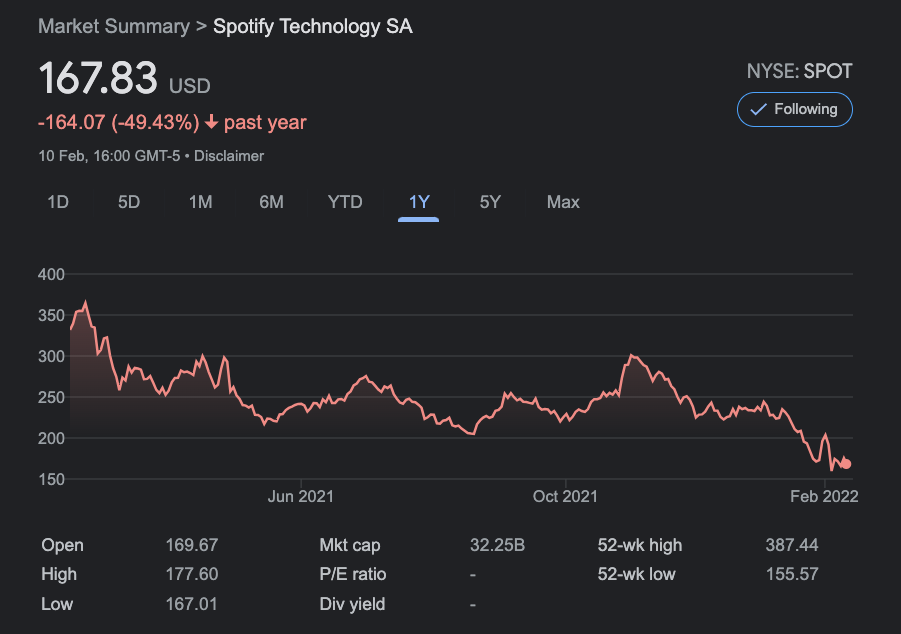This is an image of a stock summary for Spotify Technology S.A., featured on a stock market platform. At the top left corner, the label "Market Summary" appears in gray font. Directly below this heading, a large symbol followed by a right-facing arrow is displayed alongside the company's name, "Spotify Technology S.A." On the top right-hand side, the text "NYSE: SPOT" is prominently shown, with a checkmark box just below it indicating that the user is following this stock.

The current stock price is prominently listed as $167.83, situated on the left-hand side just below "Market Summary". Beneath the stock price, in smaller red font, the text reads "-$164.07" and, in parentheses, "-49.43%", both accompanied by a red downward arrow denoting a significant decline over the past year. Lastly, a timestamp at the bottom left reads "10 February 1600 hours GMT," indicating the most recent update of this stock summary.